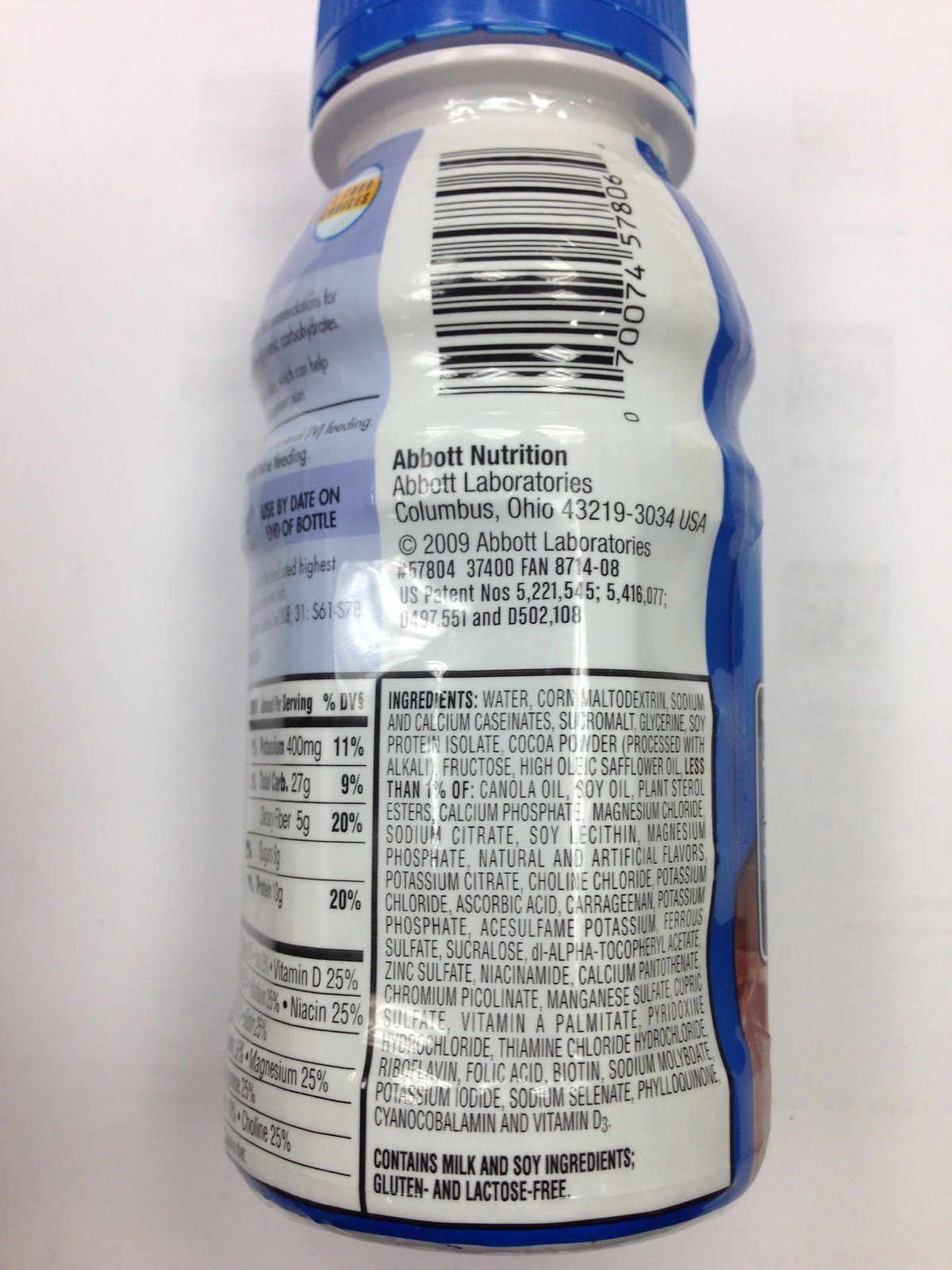The image depicts a 12-ounce protein beverage bottle from Abbott Nutrition, lying flat on a white surface with a blue plastic cap. The bottle, primarily blue with brown accents and a white labeling section, features a detailed ingredient list including water, chromodextrin, sodium and calcium caseinates, and cocoa powder. The word "INGREDIENTS" is boldly printed, followed by a comprehensible list in all caps. The back of the bottle reveals a standard black barcode, along with nutritional facts like niacin, vitamin D, and magnesium, though some values are partially obscured. Key brand details such as Abbott Nutrition, Columbus, Ohio, and a copyright date of 2009 are centrally placed. The label also includes a warning in bold black text about milk and soy contents, noting the product is gluten and lactose-free. Additionally, a white circle outlined in blue sits in the top left corner, featuring yellow blocks and black writing, although the text is not entirely legible due to the angle of the image.